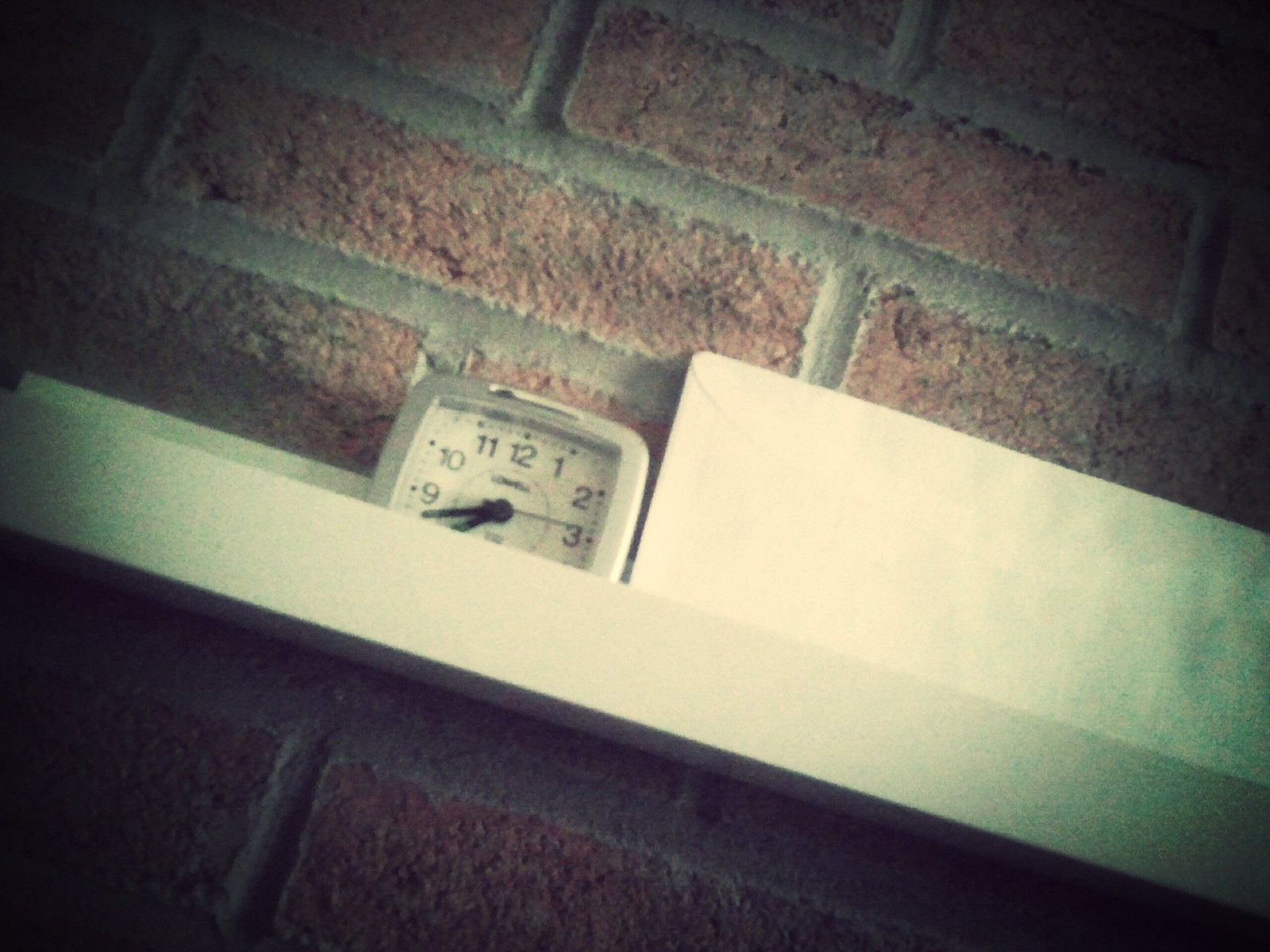The image features a close-up view of a small, portable clock that exudes simplicity and functionality. The clock's design is minimalistic, with a predominantly white dial and an equally white face, encased in a plain, white shell. Its shape is unique, resembling a squarish circle with gently rounded edges. The clock's hands and numerical markings are printed in black, providing a stark contrast and easy readability amidst the all-white backdrop. 

This compact timepiece is positioned on a ledge, with a rustic brick wall serving as the background, adding a touch of texture to the otherwise straightforward composition. Additionally, a long, white envelope is visible behind the clock, devoid of any writing or identifying marks, further emphasizing the clean and uncluttered aesthetic of the scene.